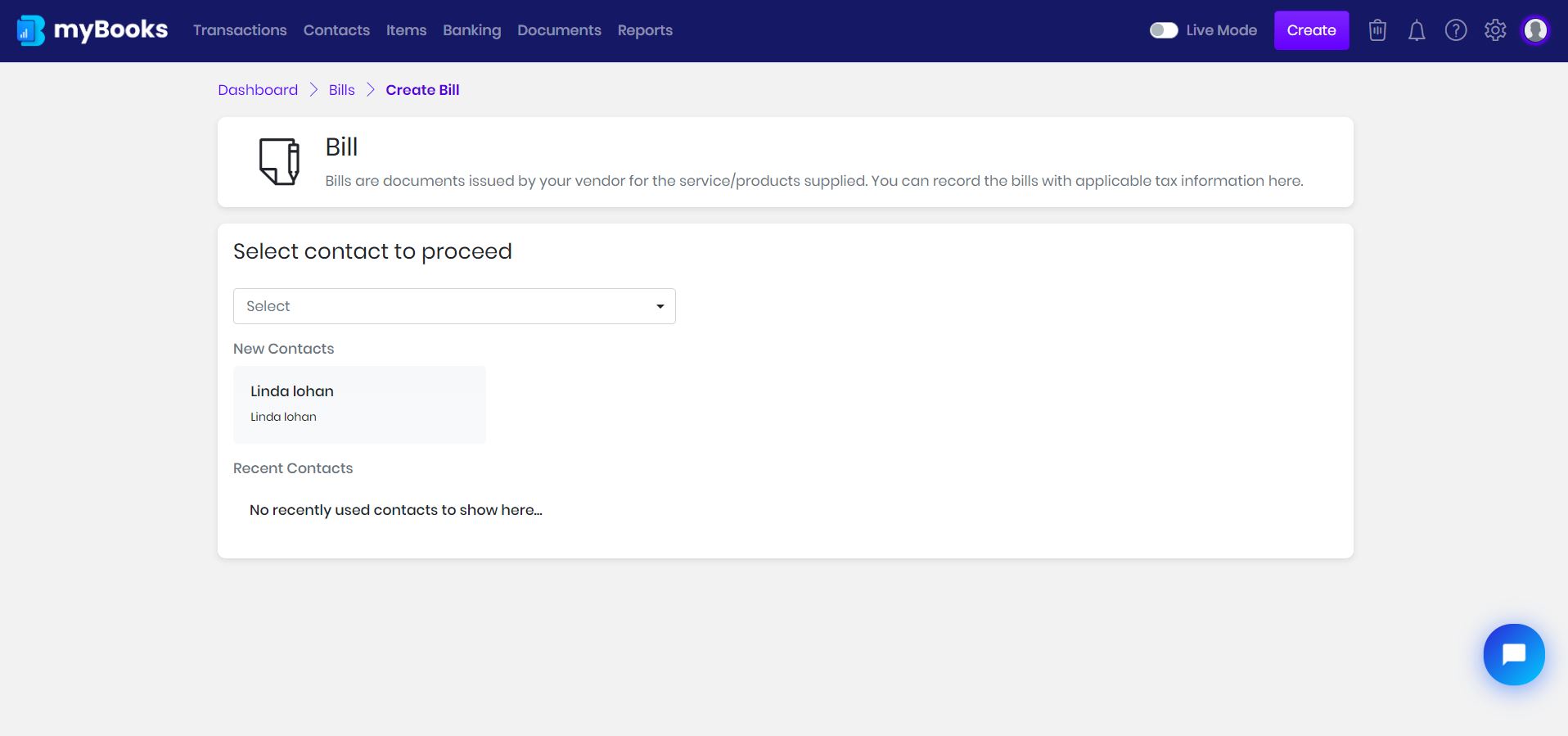The image showcases a web page titled "My Books" with the title styled as "my Books" (lowercase "m" and uppercase "B"). This title is rendered in a white font set against a blue background. To the left of the title, there's a light blue logo resembling stacked books. 

The top navigation bar features several tabs in a pale gray font: Transactions, Contacts, Items, Banking, Documents, and Reports. The background of the area beneath the top bar is a light pinkish-gray color. Centered on this backdrop is a white rectangular section.

Just above this white area, the word "Dashboard" appears in a lilac-colored font. Below "Dashboard," the words "Bills" and "Create Bill" are also in lilac, with "Create Bill" in bold. 

Within the white rectangle, there is an icon representing a bill, accompanied by the word "Bill" in a black font. The main heading within this section reads "Select Contact to Proceed," followed by dropdown bars labeled "Select." Below this section, there is an option labeled "New Contacts."